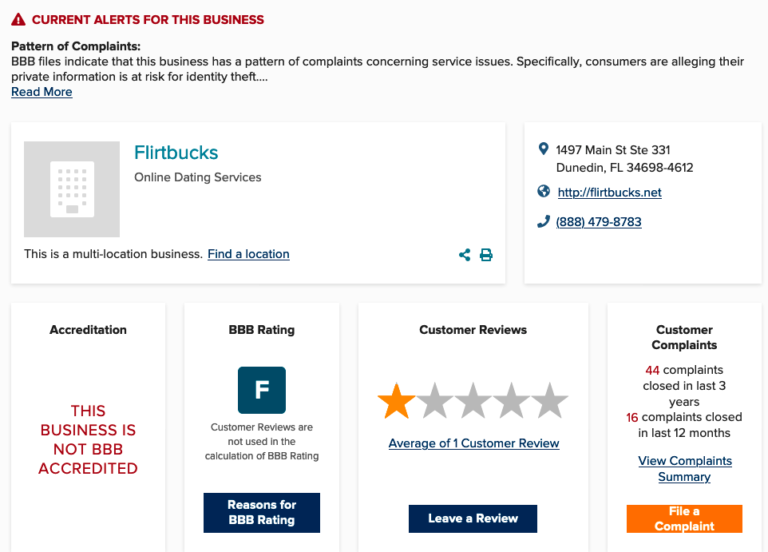**Detailed Caption: Screenshot of Better Business Bureau Alert for Flirt Bucks Online Dating Service**

This image is a detailed screenshot from the Better Business Bureau (BBB) website. At the top of the screenshot, there is a red alert triangle symbol followed by red text stating, "Current alerts for this business." Below this, bold text reads, "Pattern of Complaints," with a description indicating that the BBB has identified a recurring issue with this business. The BBB files reveal that Flirt Bucks, an online dating service, has a pattern of complaints from consumers alleging that their private information is at risk for identity theft.

A blue, underlined link labelled "Read more" provides further details. The business in question, Flirt Bucks, appears in the description along with an icon resembling an iPad within a gray field, suggesting a digital interface. It is noted that Flirt Bucks is a multi-location business, with a dedicated section for finding specific locations. Key contact information is listed as follows: 14987 Main Street, Suite 331, Dunedin, Florida, 34698-4612, with the website http://flirtbucks.net and a phone number 888-479-8783.

To the right side of this information, there are buttons for sharing and printing the page. Underneath this section, the screenshot shows four main categories related to the business: Accreditation, BBB Rating, Customer Reviews, and Customer Complaints.

Highlighted in red, the text indicates that this business is not BBB accredited and holds an F rating. It notes that customer reviews are not factored into the BBB rating, and a blue button is available for users to see the reasons behind the BBB rating. The customer review section shows an average rating of one star from a total of one review, with a "Leave a Review" button available for additional feedback.

In the Customer Complaints section, it is noted in red that there have been 44 complaints closed in the last three years, with 16 of those complaints closed in the past 12 months. A text link is provided for viewing a summary of the complaints, along with an orange button for filing a new complaint.

Overall, the screenshot provides a comprehensive overview of the BBB's assessment and consumer feedback for the Flirt Bucks online dating service.